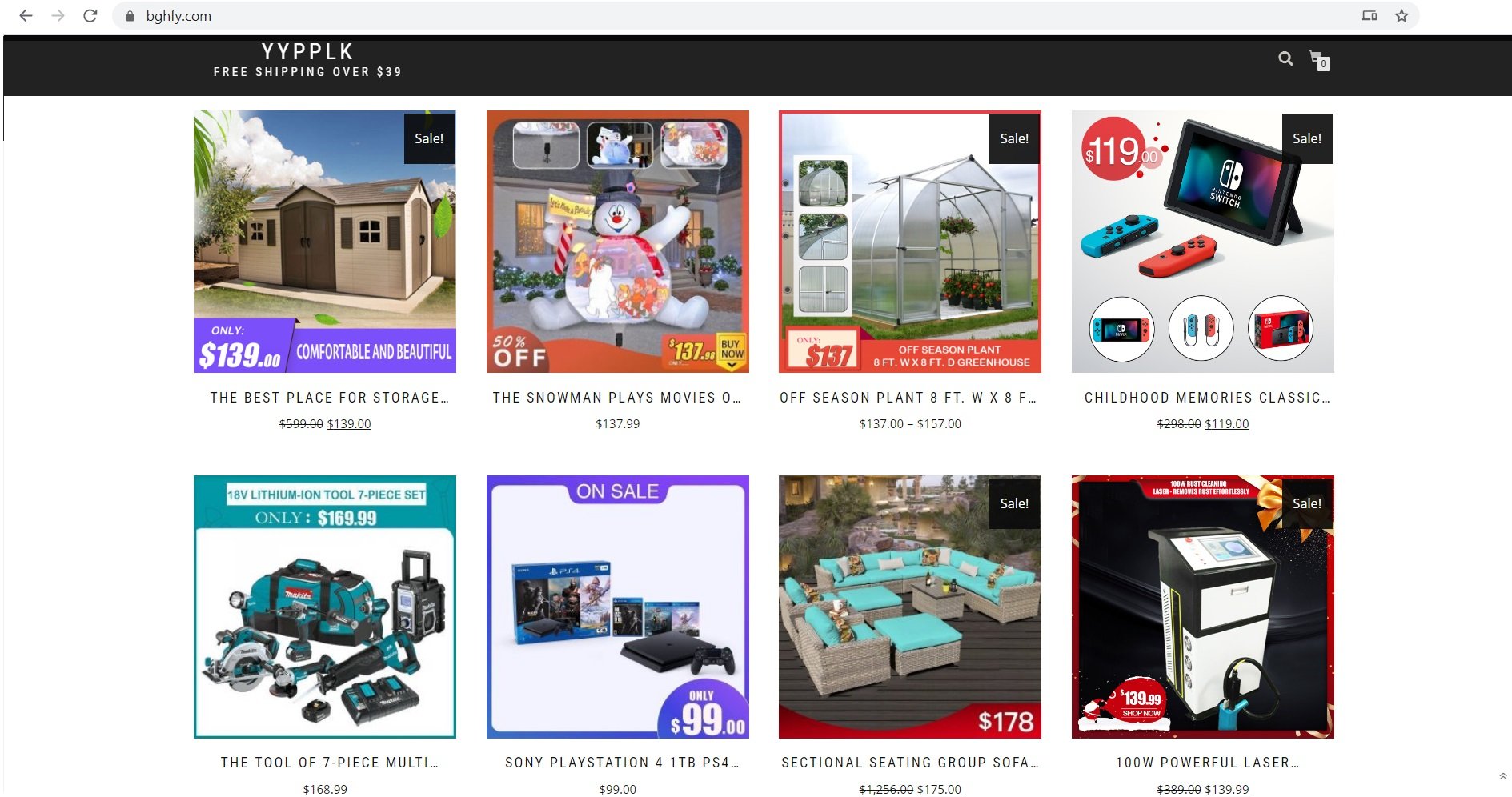This screenshot features a black banner at the top with white text reading "YYPPLK". Beneath this, it offers "Free shipping over $39". On the right side of the banner, there is a search icon and an empty shopping cart.

Below the banner, there are two rows of square images, each showcasing a different product:

- **First Row:**
  1. **Storage Unit**: A structure priced at $139 with a central door and two sets of windows on each side.
  2. **Snowman Projector**: An orange box displaying a snowman with a transparent belly playing the movie "Frosty the Snowman". The item is offered at a 50% discount, costing $137.99.
  3. **Greenhouse**: An 8x8 feet outdoor plant greenhouse priced between $137 and $157.
  4. **Nintendo Switch**: A console priced at $119, featuring blue and red Joy-Con controllers, labeled with "Hunt childhood memories classic".

- **Second Row:**
  1. **18V Lithium-ion Tool Set**: Presented in a turquoise box, it includes 27 pieces and sells for $169.99.
  2. **Sony PlayStation 4**: A purple-edged square denotes this 1-terabyte console on sale for $99.
  3. **Outdoor Sectional Seating**: A wicker patio sofa with turquoise pillows, priced at $178, described as a sectional seating group sofa.
  4. **Laser Printer**: Priced at $139, highlighted for its powerful 100-watt laser capability.

Each product image is detailed, providing potential buyers with clear information and pricing.